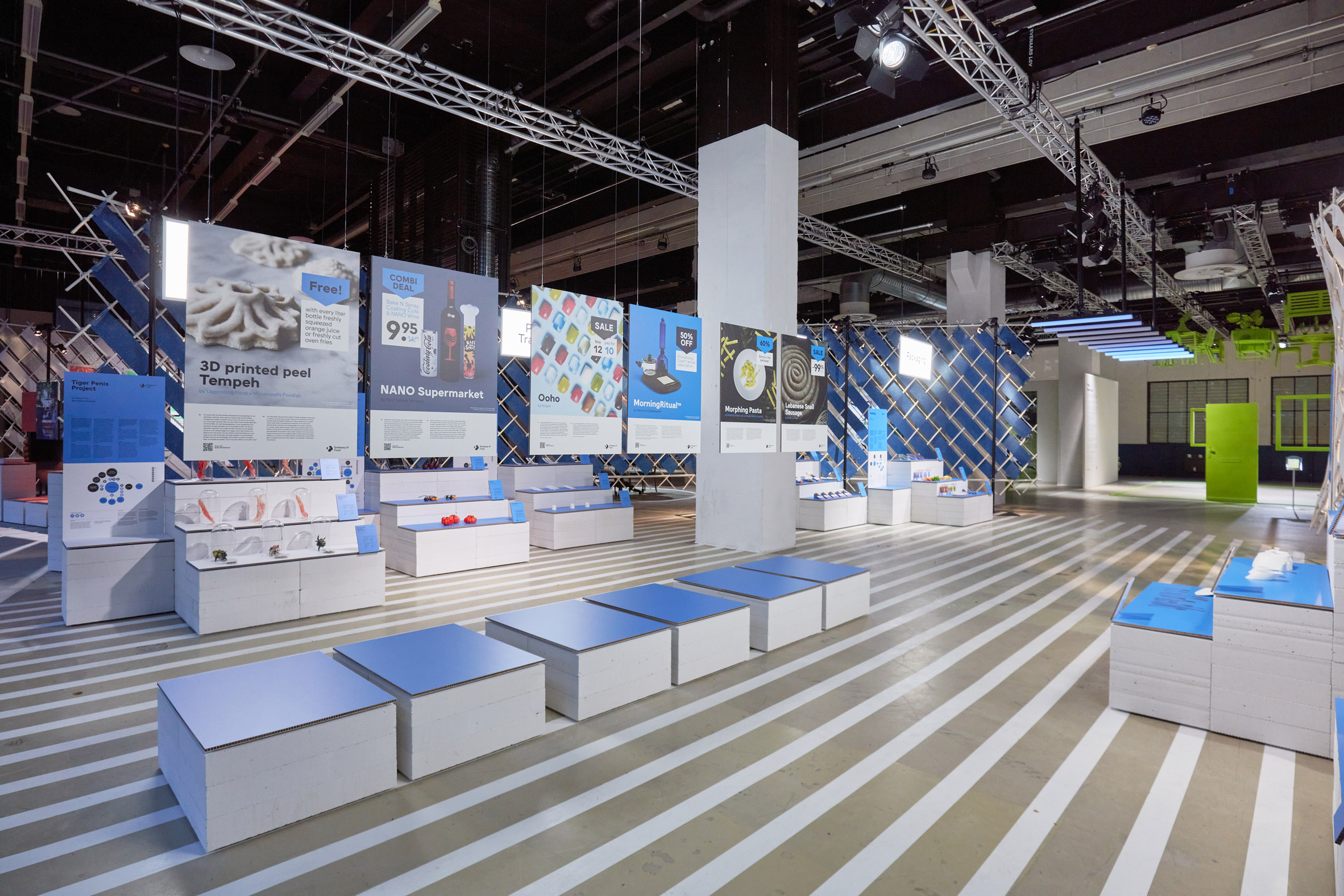The image showcases a large, open indoor convention center with a high ceiling supported by a visible metal framework, adorned with spotlights and other lighting fixtures. The floor features a concrete surface interspersed with white and gold stripes. Scattered throughout the area are numerous white and blue booths, platforms, and block-like seating arrangements. The scene is bustling with people, spaced equidistantly across the space. Various backdrops and poster boards displaying advertisements, including identifiable ones for "3D Printed Peeled" and "Nando Supermarket," hang from the walls and ceilings. Towards the middle right of the image, a green door and green metal framework contrast with the predominant blue and white color scheme. A central pillar surrounded by poster banners adds to the organized yet vibrant atmosphere.